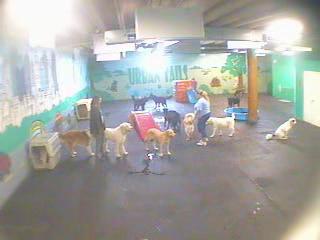The image appears to be a low-quality, grainy photograph, seemingly captured from a security camera in a possible basement setting. The room's floor is dark concrete, and the walls are painted in a mix of turquoise and grass green. A mural on the back wall, depicting an outdoor scene with trees and possibly a beach, prominently features the words "Urban Tails." 

The scene is bustling with activity, reminiscent of a dog obedience class or a doggy daycare. There are at least ten dogs of various breeds spread throughout the room, some gathered in the middle and others scattered towards the foreground. Two women are present, engaging with the dogs: one with a white dog at her side standing to the left, and another with blonde hair in a blue shirt, accompanied by two additional white dogs, standing nearer to the center. The room also contains a few large dog crates, a baby pool, a slide, and other dog activity equipment, indicating a space designed for canine care and training. The overall impression is one of a lively, yet somewhat chaotic environment tailored for dogs amidst everyday human interaction.